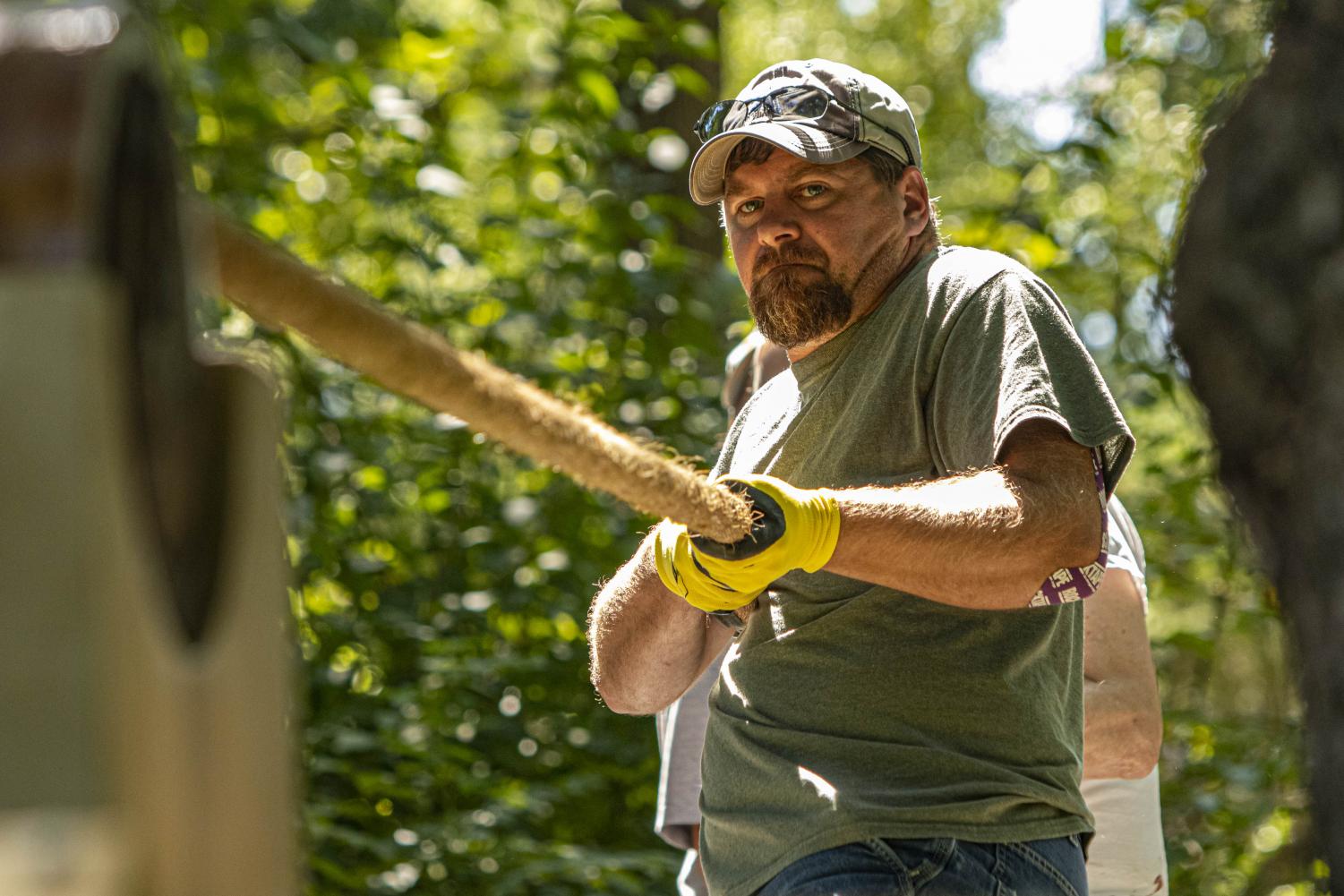The outdoor photograph features a bearded man with brown hair, wearing a green short-sleeve shirt and blue jeans. His tan complexion and arm hair are visible, and he sports a maroon and white bandage on his right elbow. He is also seen in a beige baseball cap adorned with sunglasses on top. The man, who has bright yellow gloves on, is intently pulling a thick yellow rope, potentially in a tug-of-war contest or work-related activity. His facial expression shows determination, and there is a hint of someone else behind him, identifiable only by their elbow. The background includes trees and brush, adding to the impression that the scene is taking place in a semi-rural or wooded area. The photo, taken horizontally, captures the dynamic effort and teamwork in the moment.